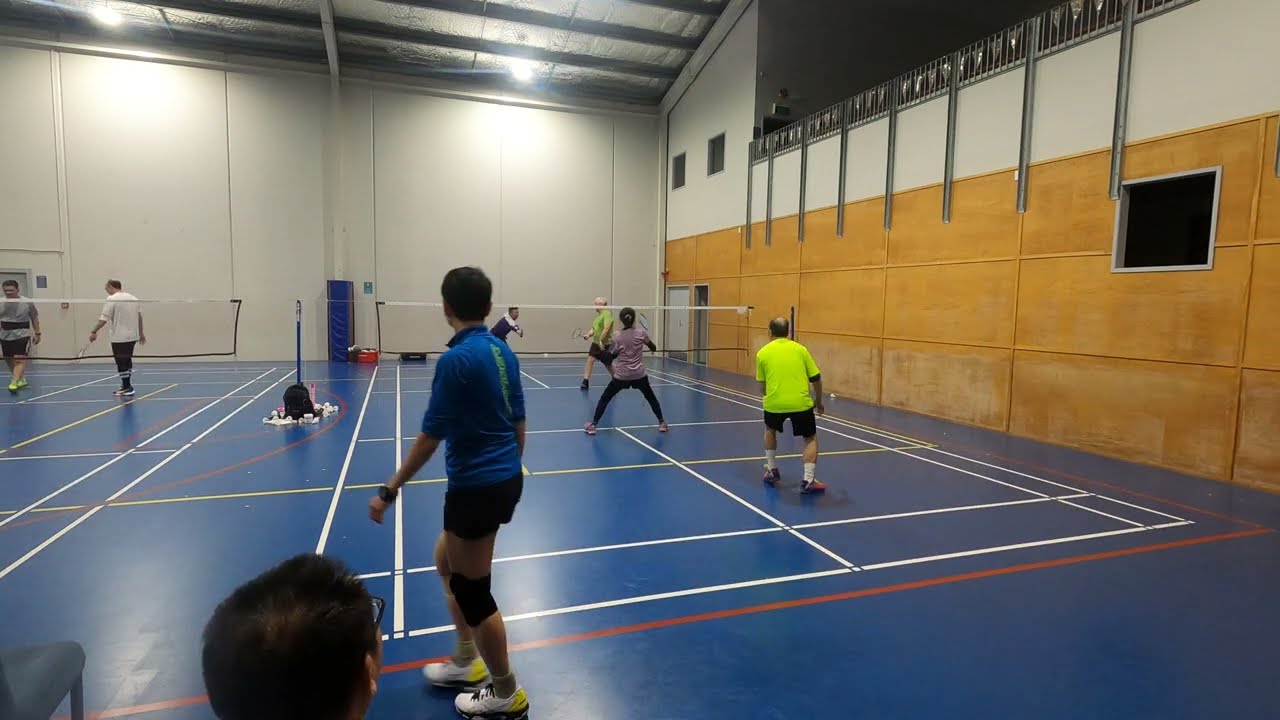In this vibrant image of an indoor gymnasium, a lively game of badminton is in progress, occupying a prominently blue court marked with white, yellow, and red lines. High, exposed beams line the ceiling, which soars over 20 feet above the players, contributing to the bright, well-lit environment. The gym features eggshell-white walls and brown paneling on the right side, creating a spacious and well-maintained venue for indoor sports.

The scene depicts a fast-paced game with a net stretched across the court, akin to a volleyball net, which separates the players. On the near side, three players—one holding a racket—are engaging in the match, donned in colorful shirts and shorts, with one woman notably wearing tights. Across the net, two players are intensely focused on the game. To the left, another court is partially visible, also bustling with activity.

A small station in the middle of the courts contains a collection of shuttlecocks, suggesting multiple games are either ongoing or in preparation. The vibrant setting, complete with overhead lighting, ensures that the matches are well-illuminated, making this a perfect venue for an energetic game of badminton.